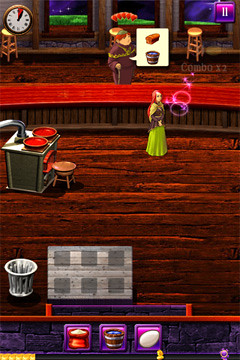In this image, reminiscent of a still from a video game with a portrait orientation, the scene is set in a medieval bar. The focus is on a woman behind the bar, presumably the barkeep, who appears to be taking an order from a customer dressed in a regal, purple robe that resembles a pope's attire. Behind this customer, a series of barstools are lined up against the bar. The setting features a rudimentary cooking station with a stove and three available ingredients: a red sack of flour, an old wooden bucket filled with water, and a single egg. The customer seems to be requesting a loaf of bread along with the bucket of water, adding a touch of medieval realism to the cooking game environment.